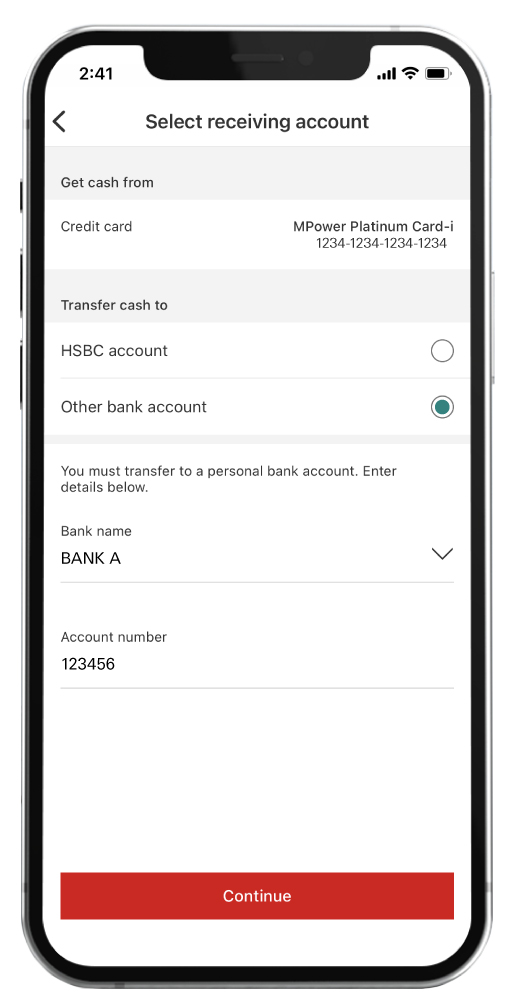The image displays a vertically oriented cell phone with a sleek, silver-colored bezel that wraps around its edges, reflecting light with a glossy finish. On the left side of the phone, there are three protruding buttons, while the right side features a single, slightly indented button. The interior of the screen is framed by a slim black border, which slightly widens at the top where a speaker and camera are located.

At the top-left corner of the screen, "2:41" is displayed against a white background, indicating the current time. The top-right corner shows a nearly full battery icon along with full signal and Wi-Fi indicators.

The screen's main interface displays a financial transaction application. The prompt reads "Select Receiving Account," accompanied by options to navigate back or access more information. The user is instructed to "Get cash from Credit Card" using a specific card identified as "mpowerplatinumcard-i1234-1234-1234-1234." The user can transfer cash to an HSBC account or another bank account, with "Other Bank Account" being selected.

Below, the interface requests bank account details, including fields for "Bank Name" and "Account Number," with "123456" filled in for the account number. A prominent red "Continue" button is positioned at the bottom of the interface, prompting the user to proceed with the transaction.